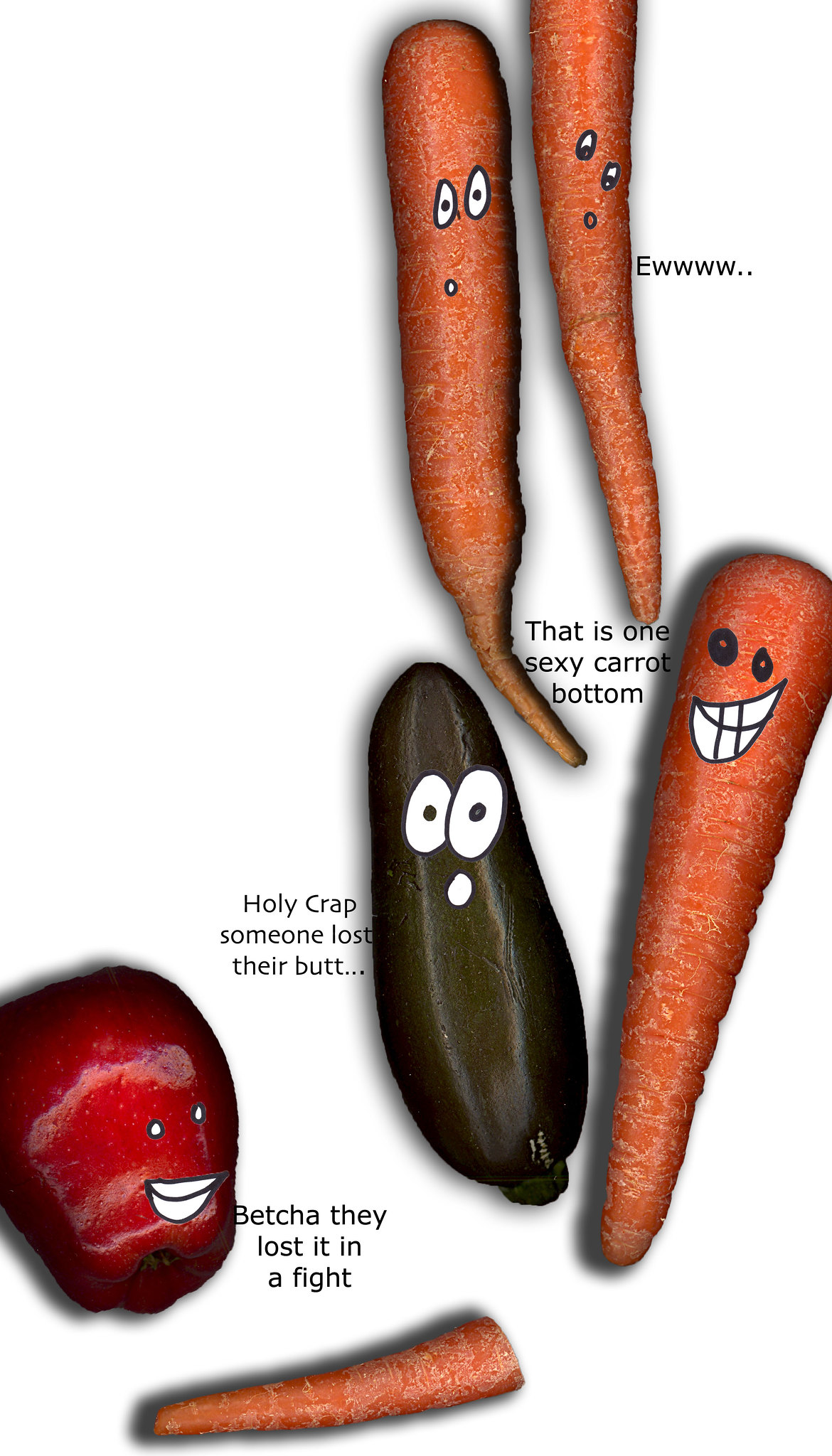In this quirky, illustrated image set against a plain white background, a humorous scene unfolds featuring various anthropomorphic vegetables and a fruit. At the top right, two carrots display surprised expressions, accompanied by black text reading "EWWWWW..." Below them, another carrot grins mischievously with a caption that reads, "That is one sexy carrot bottom." A black cucumber to the side, bearing a shocked face, exclaims, "Holy crap, someone lost their butt." Near the bottom, a red apple adds to the humor with the line, "Betcha they lost it in a fight," alluding to the severed carrot piece at the very base of the image. Each character has a simple face drawn on it, giving them distinct personalities and enhancing the overall comedic effect.